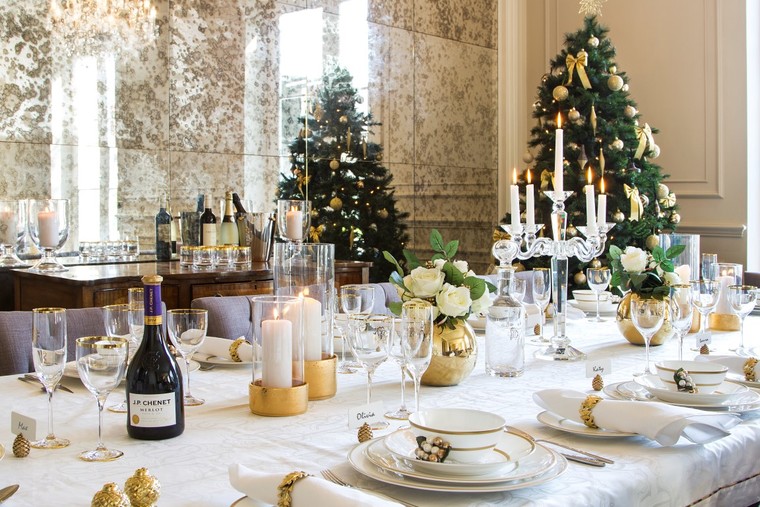This photograph captures an opulent and festive dinner setting, prepared with meticulous detail for what appears to be a Christmas celebration. At the centerpiece of this grand banquet hall is a long, white-linen-covered table, resplendent with luxurious place settings, each featuring a large plate, a smaller plate, a soup bowl, a salad bowl, and possibly an additional dish. The plates are white with gold accents, complemented by neatly rolled white napkins encircled with gold bands. Sparkling wine glasses and water glasses are positioned at each setting.

The table is adorned with a stunning array of decorations, including two large gold-colored vases brimming with white roses and green leaves. Tall white candles in clear glass cylinders run along the center, surrounded by additional crystal candelabras, each hosting long white candles. Each place setting is marked by a name card, held in an elegant golden pine cone clip, underscoring the festive ambiance.

The room itself adds to the grandeur, with high ceilings inferred from the tall Christmas trees illuminated in the background. One tree, adorned with orange ornaments, stands centrally, while another off to the right showcases ribbons and silver and gold decorations. The walls vary from shiny beige and black-speckled stone to French-inspired whitish beige panels, enhancing the sophistication of the space.

In the foreground, a bottle of champagne labeled J.M. Chaney, wrapped in gold foil, hints at the evening's indulgence. Behind the table, a bar area with a marble top and wooden base displays an assortment of liquor bottles and glasses, ready for the evening's festivities. The bar and the surrounding marble or stained glass paneling complete this exquisite dining scenario that is yet to welcome its guests.